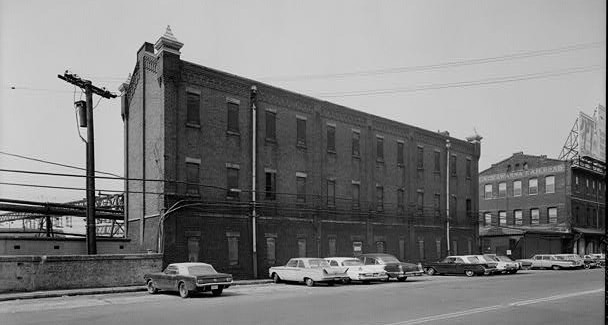This black-and-white photograph captures a large, rectangular, three-story industrial building made of small rectangular bricks. The flat roof with tall brick pillars at the ends accentuates the building's early 20th-century architecture. Even rows of horizontally aligned rectangular windows with black casements punctuate each floor, giving the structure an organized, almost factory-like appearance. In front of the building lies a light-colored asphalt road with double lines running diagonally from the bottom center to the top right corner. 

A paved parking lot, populated with vintage cars from the late 1950s or early 1960s—typically large sedans—lines the road. To the building's left, a T-shaped wooden utility pole, equipped with a transformer, extends multiple black wires towards the right side of the image. Adjacent to this utility pole is a low brick wall. In the background, an elevated train track further enhances the industrial setting. 

On the right side of the photograph, another three-story industrial building with a peaked roof features prominently. This building has a large wooden latticework holding a billboard with multiple lines of text. The scene is bathed in a grayish light typical of black-and-white imagery, with the reflection on the tops of the parked cars suggesting a clear, sunny day.